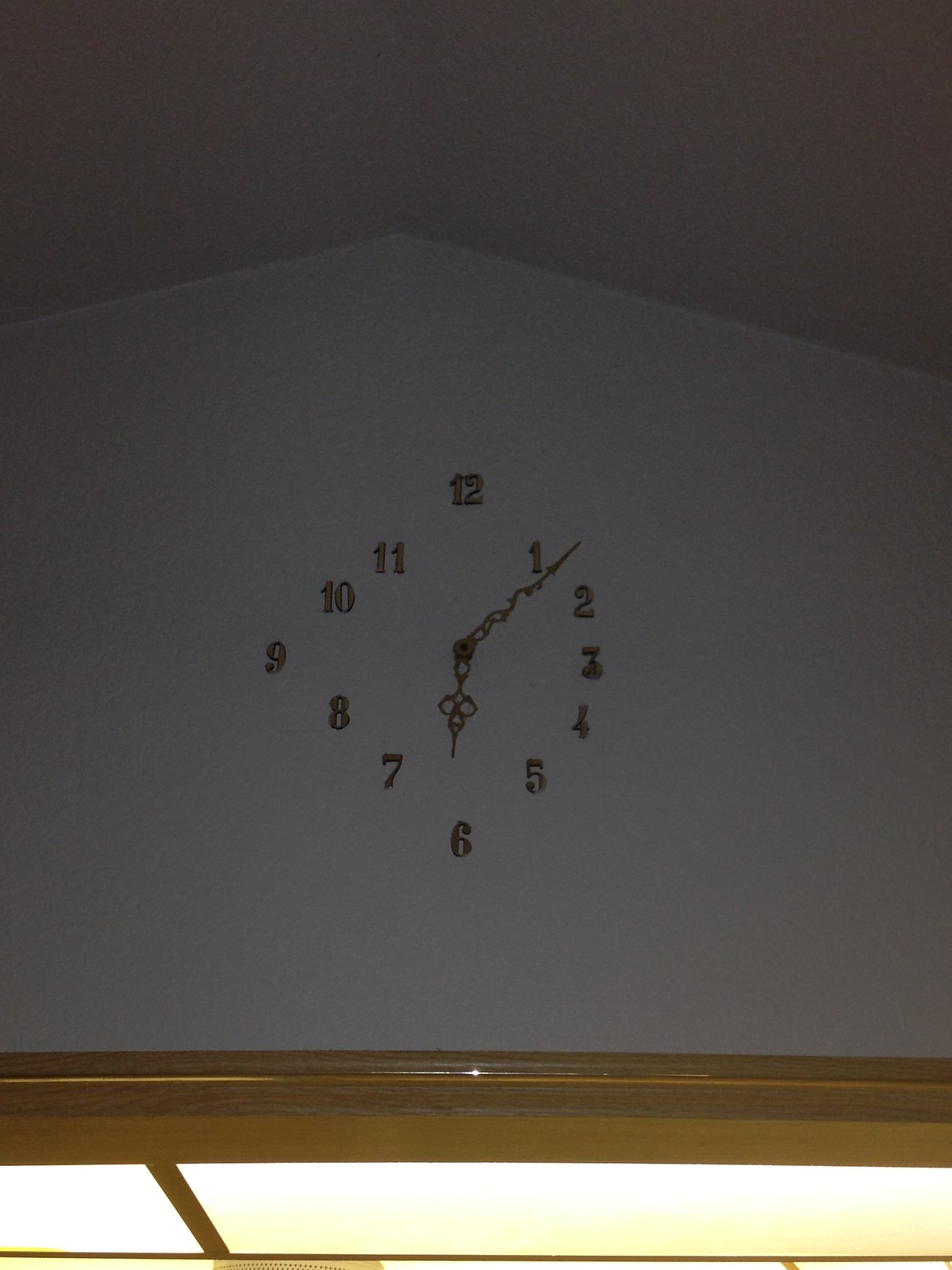This is an indoor photograph of a highly unusual and intriguing clock on a white wall in dim lighting. The clock doesn’t have a traditional frame; instead, gold metal numbers are affixed directly to the wall in sequential order. The arrangement deviates from a perfect circular pattern— the right half appears round while the left half resembles a diamond shape. Notably, the positions of the 12 o’clock, 6 o’clock, and 9 o’clock numbers are slightly off, whereas the 3 o’clock number aligns correctly within the sequence. In the center, bolted to the wall, are the minute and hour hands, but there is no second hand. The clock is positioned high on the wall, with a wooden beam below it marking the beginning of the ceiling composed of panels containing fluorescent lights, which illuminate the space. The unusual shape of the ceiling panels converges at a point, adding another layer of interest to the image. According to the clock, the time seems to be around 6 or 7 o'clock.